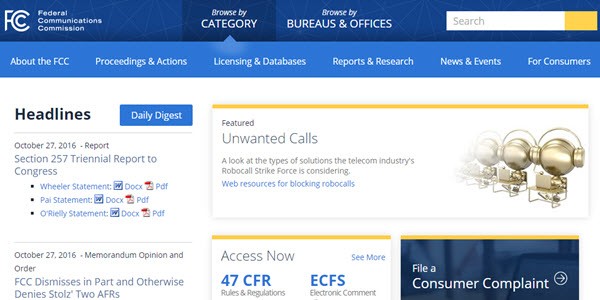This screenshot captures the homepage of the Federal Communications Commission (FCC) website. The website features a prominent navigation bar at the top, which is either black or blue, displaying the FCC logo on the upper left-hand corner. Directly to the right of the logo are the main navigation options: "Browse by Category" and "Browse by Bureaus and Offices."

Beneath this navigation bar are additional sub-menus that include: "About the FCC," "Proceedings and Actions," "Licensing and Databases," "Reports and Research," "News and Events," and "For Consumers." In this screenshot, the "Browse by Category" tab is highlighted, though no submenu options are currently selected.

The main content area of the webpage is focused on providing information regarding unwanted calls. It details how consumers can report these unwanted calls to the FCC, offering guidance on steps to take and resources available for assistance.